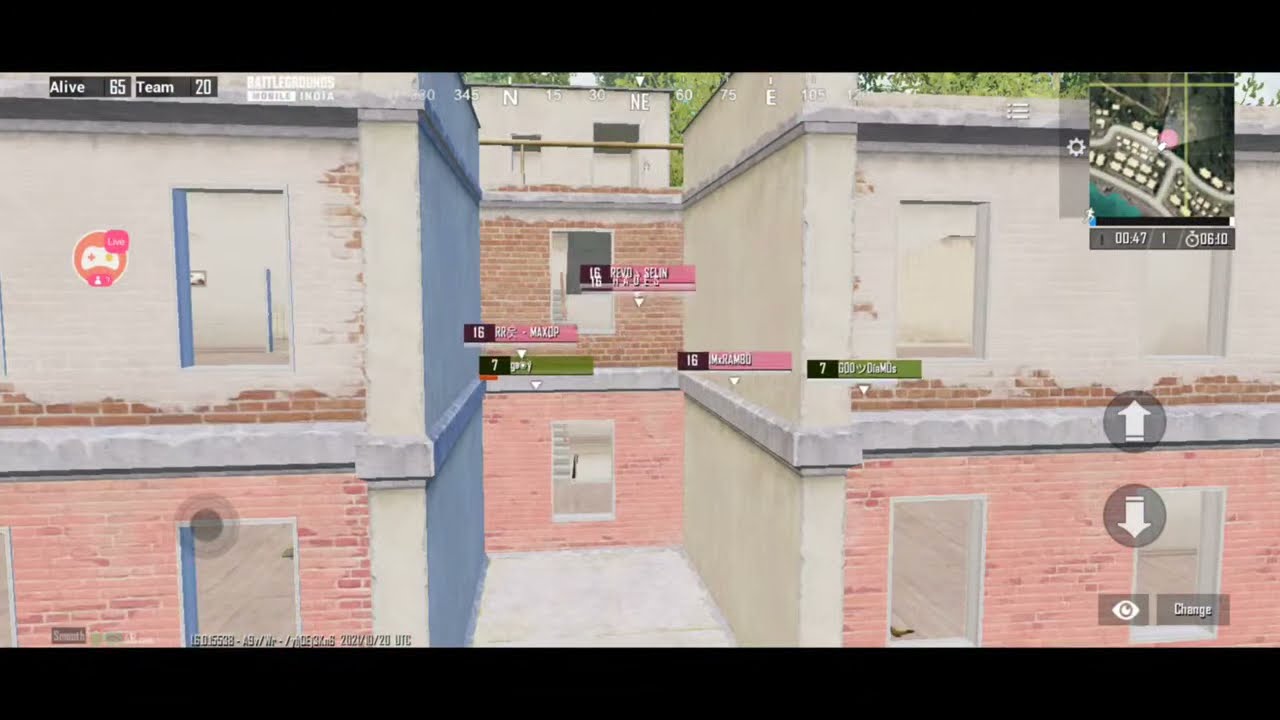The image depicts a detailed, immersive interface from a video game, showcasing an exterior view of buildings split by a narrow alleyway. The building on the left boasts a facade of brown, white, and pink bricks with two doors, one on the upper level and one on the lower level. This structure features a blue outer wall. To the right, another building mirrors this design, constructed with the same white, brown, and pink bricks, and includes windows on both levels. Between these two, a narrow road leads to another brick building in the background, with its upper level clad in brown and the lower in pink, each level also hosting windows. The screen is filled with elements typical of a game: small rectangles indicating player usernames and numbers are scattered across the buildings, an eye icon in the bottom right with "Change" next to it, and a mini-map in the upper right. Additionally, "Alive 65, Team 20" is prominently displayed in the upper left corner, resembling a sports score layout. The road in the alley appears to be of gray concrete, creating a clear path through this engaging virtual environment.